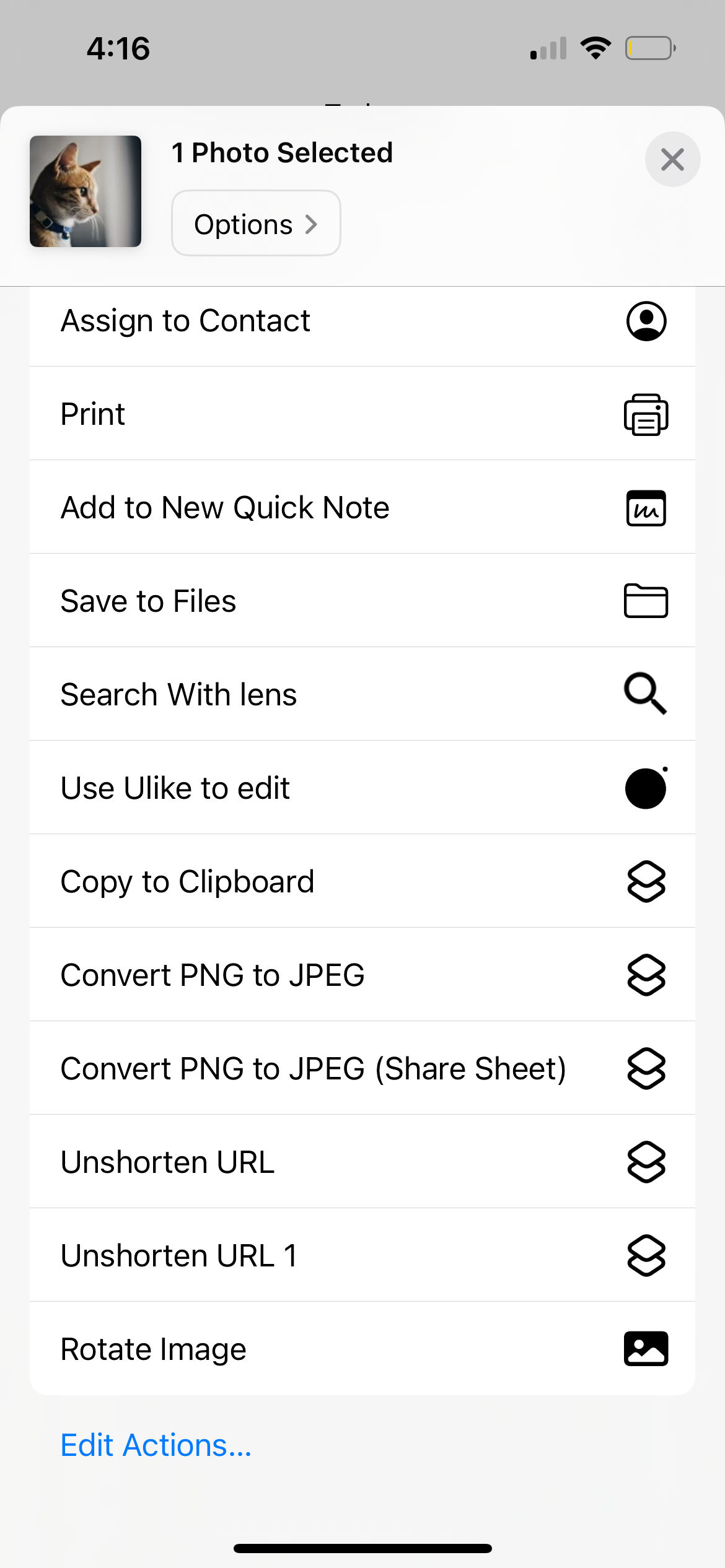The image is a rectangular vertical screenshot of a cell phone screen, with no visible physical phone. The background of the screenshot is primarily white. At the top, there's a grey bar displaying the time, which is 4:16, alongside connectivity information: one out of four bars of cell tower strength, full Wi-Fi signal, and a low battery level. 

Below this, a brown and white cat avatar is shown facing right, under the header "One Photo Selected" with an accompanying options arrow directing to the right. The menu lists various actions that can be taken with the selected photo:

1. Assign to Contact
2. Print
3. Add to New Quick Note
4. Save to Files
5. Search with Lens
6. Use U-Like to Edit
7. Copy to Clipboard
8. Convert PNG to JPEG (twice, with the second instance in brackets indicating it is from the share sheet)
9. Unshorten URL (listed twice, with a slight difference as the second instance is labeled Unshorten URL1)
10. Rotate Image

At the bottom of this list, there's a blue option labeled "Edit Actions." 

The overall context of the screen suggests that the user has selected a photo of a cat and is being prompted to choose an action for the image within what appears to be a settings or options page.